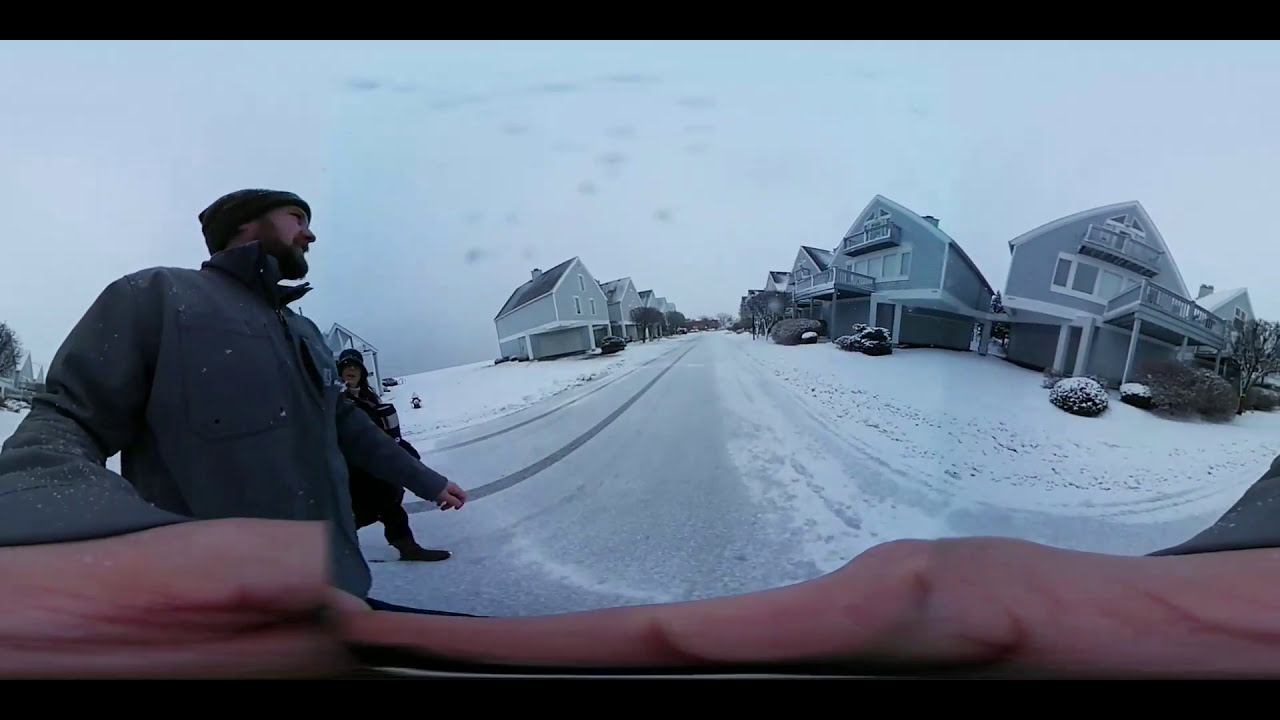The panoramic, warped image showcases a suburban neighborhood blanketed in snow after a recent snowstorm. The 360-degree camera perspective distorts the view, making the scene appear curvy and angular. The foreground prominently features a man on the left side wearing a black beanie and a dark gray jacket, with his hand stretched outwards, dominating the bottom part of the image. His fingers appear elongated due to the wide-angle lens. A woman stands next to him, dressed warmly in a thick coat and a wide-brimmed hat, carrying a bag beneath her arm. The snowy road leads towards rows of almost identical houses positioned on both the left and right, each with a gray exterior, white framing, and dark gray or black pointed roofs. The houses feature large porches, some appearing to be on stilts, with upper levels adorned with numerous windows. Despite the overcast and monochromatic scenery, the details of suburban architecture and the freshly fallen snow create a serene yet surreal winter landscape.